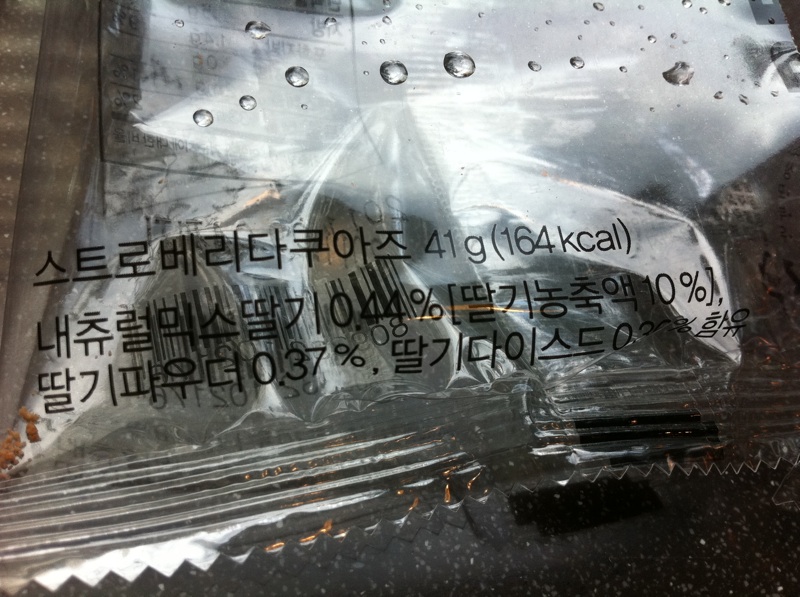A detailed close-up of a clear plastic bag, likely designed to contain snacks such as potato chips, occupies the frame. The bag exhibits some moisture, evident by the beads of water clinging to its surface. Through the transparent material, a nutrition label on the back is partially visible. The front of the bag features text, which appears to be in either Chinese or Korean, contributing to the mystery of its contents. The only readable element in English is the weight indication: "41 grams." The image emphasizes the bag's texture and detail, capturing the viewer's curiosity about the snack it holds.